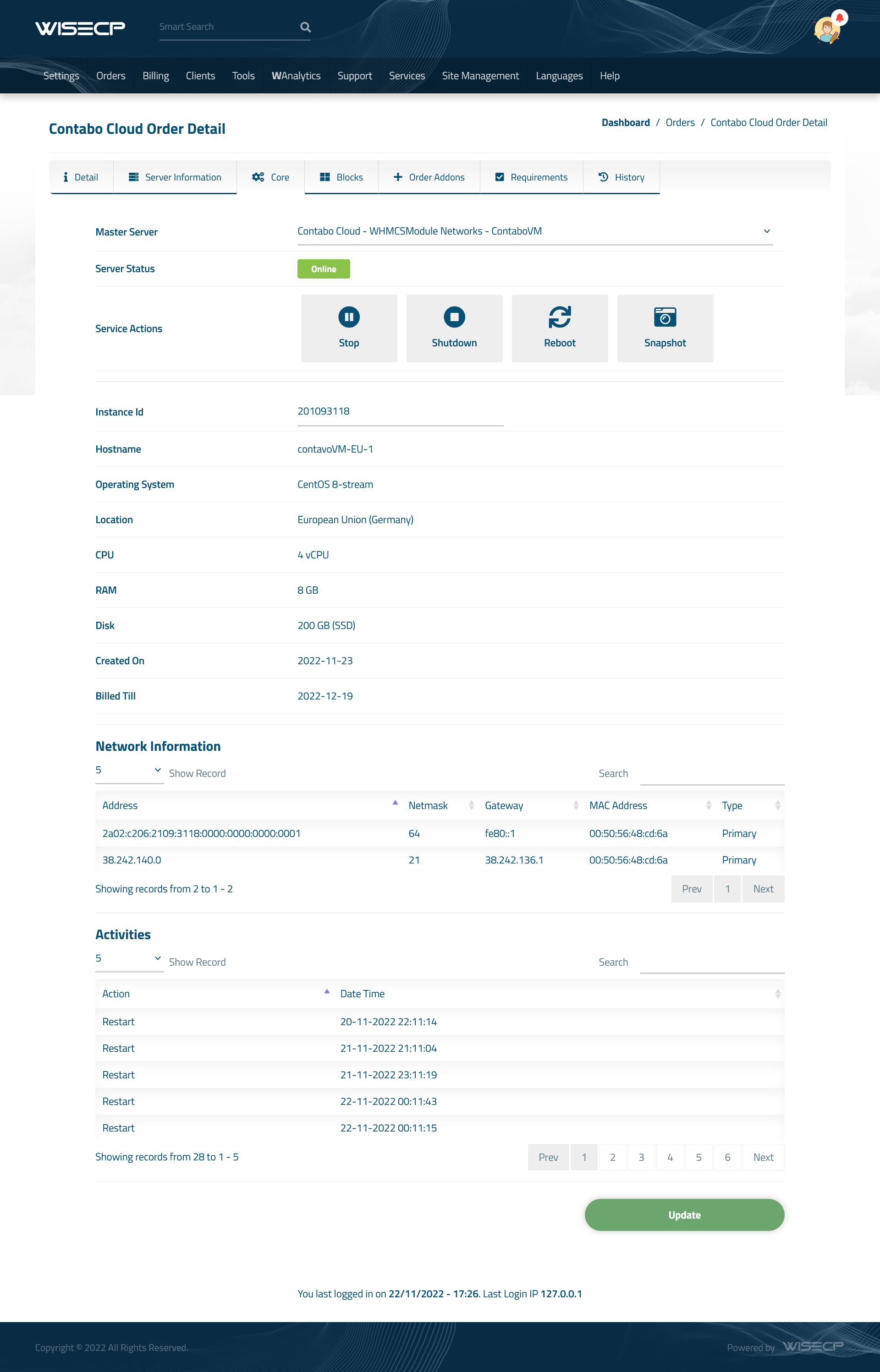Image Description:

The image showcases the homepage of WISECP, a technology-oriented website. At the top left, the WISECP logo prominently appears, followed by a search bar directly beside it. On the far right, there is a small circular profile picture of a young girl, which features a red mark that could potentially be a lock icon.

Directly beneath the WISECP logo are several menu items in capital letters, albeit in a very small font. These include 'Settings', 'Orders', 'Billing', 'Clients', 'Support', 'Services', 'Help', and 'Languages'. Below these menus, there is a section titled "Contabo Cloud Order Detail" displayed in blue text. To the right of this title, a breadcrumb trail reads "Dashboard / Orders / Contabo Cloud Order Detail."

Further down, a row of labels reads "Master Server", "Server Status", "Service Actions", "Instance Of", "Host Name", etc. Adjacent to this row is the designation "Contabo Cloud WISECP Network / Contabo / M."

Below this section, there are four distinct action boxes. Each box has a specific function and accompanying icon: 
1. 'Stop' with a pause icon.
2. 'Shutdown' with a circle containing a white box.
3. 'Reboot' with a recycling icon.
4. 'Snapshot' with a camera icon.

The overall layout presents an organized view of WISECP’s interface, featuring user profile information, navigation menus, and server management options.